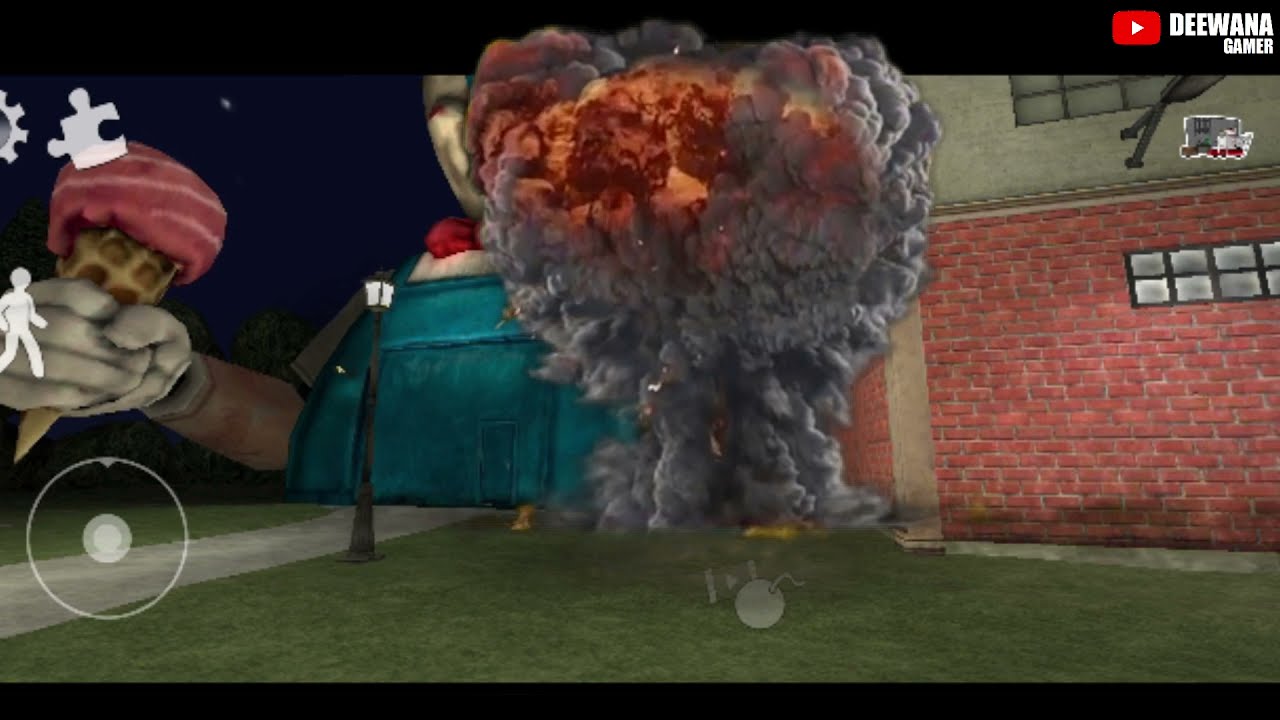The image appears to be a high-definition animated screencap from a video game. At the center, there is a dramatic mushroom cloud explosion, with a gray plume that swells into a reddish-brown top. The explosion is set against a backdrop of a red brick house, featuring a light blue, rounded structure that might be a garage, positioned to the left. A beige second story of the house is partially seen behind the blue structure. Additionally, there is a robotic arm extending from this turquoise structure, holding an ice cream cone with a whimsical face bearing a mustache and a red-striped hat, making the ice cream appear as though it's strawberry-flavored. In the foreground, a green lawn is visible, with a concrete pathway adorned by a black street lamp with a white light. The scene takes place at night against a navy blue sky sprinkled with a few stars. On the top right corner of the image, the YouTube logo is displayed alongside the username "DEEJANA Gamer" in white lettering with a black band across the top.